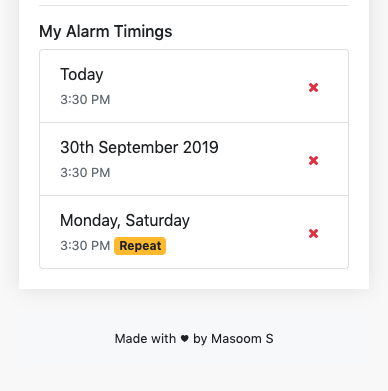This screenshot appears to be from a digital alarm clock application, possibly on a smartphone or computer. The simple user interface features a clean, white background with subtle gray tones. Prominently displayed is the headline "My Alarm Timings," indicating it is a list of the user's set alarms.

Three alarms are visible in the screenshot, each marked by a red 'X' icon for deletion. The first alarm is set for today at 3:30 PM. The second alarm, scheduled for 3:30 PM on September 30, 2019, suggests that the screenshot is several years old. Lastly, there is a recurring alarm set for 3:30 PM every Monday and Saturday.

The interface does not appear to offer additional settings such as different alarm tones, reminder texts, or customization options beyond the basic on/off functionality and the ability to delete an alarm by clicking the red 'X'.